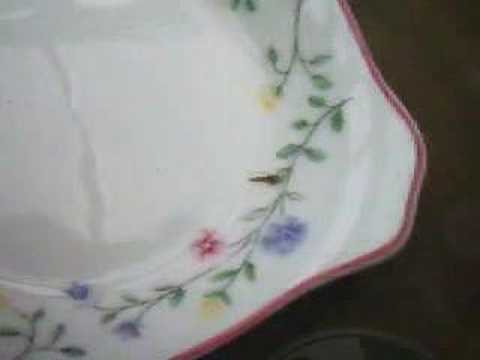This image depicts a shiny, white porcelain serving platter taking up most of the top left corner of the frame. The platter, sitting on a brown wooden surface, features a red border along its slightly angular square edges. Intricately designed, the platter showcases green stems adorned with a variety of colorful flowers, including red, yellow, blue, purple, and possibly pink blossoms. The reflective sheen of the ceramic material accentuates the vibrant floral detailing, contrasting against a dark background. The setting hints at either a cozy kitchen or a dimly lit restaurant ambiance, devoid of any text or inscriptions. The overall scene is slightly blurry, adding a touch of mystery to the delicate beauty of the platter.